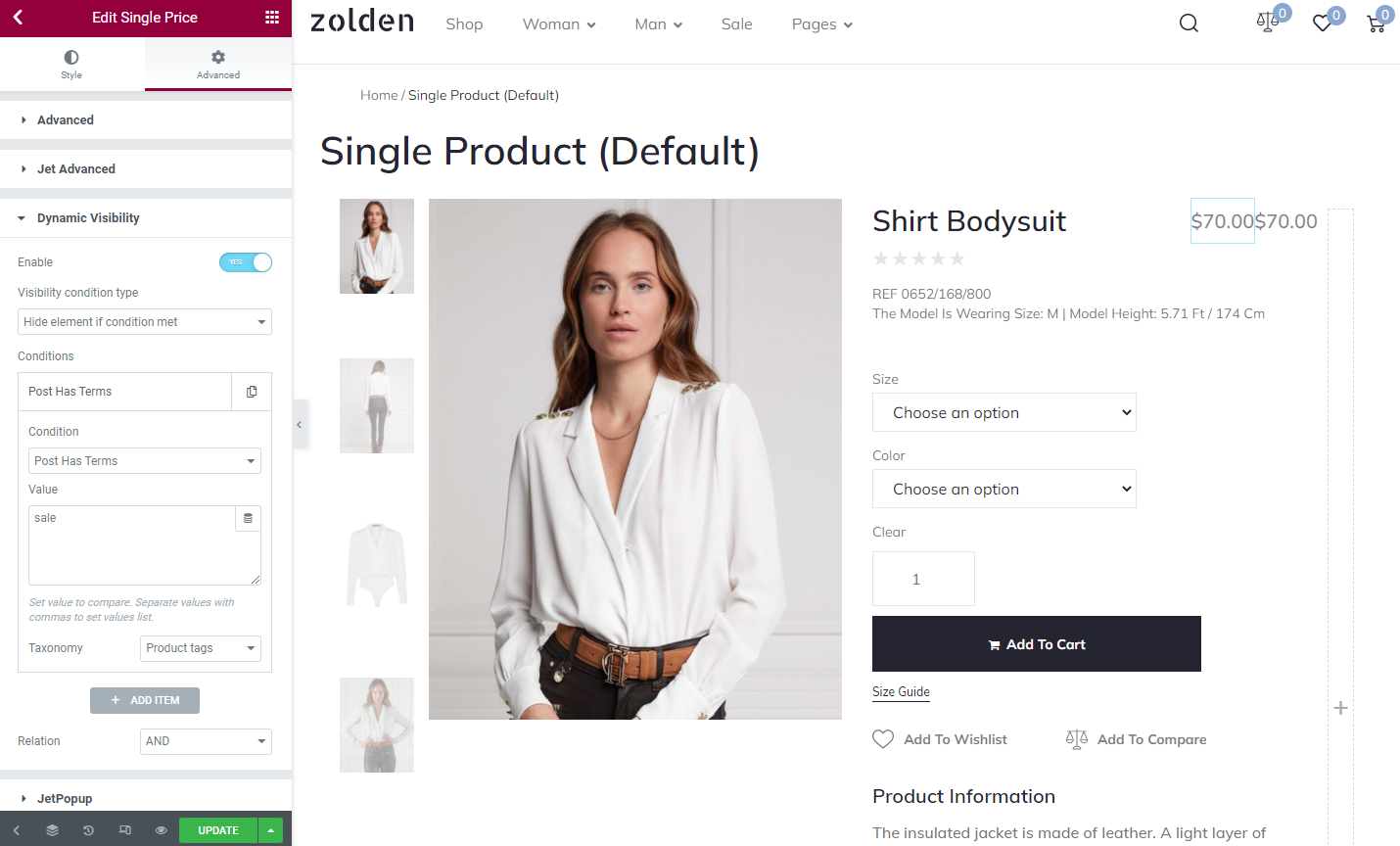This photograph captures a detailed view of an e-commerce fashion website called "Zolden" through the perspective of a logged-in administrator engaged in editing the site. At the top of the site, Zolden's simple, lowercase text logo is prominently displayed. Adjacent to the logo, the main menu options are listed, reading: "Shop," "Woman," "Man," "Sale," and "Pages." In the upper right-hand corner, there are icons for Search (magnifying glass), Compare (scales), Favorites (hearts), and the Shopping Cart; all the indicators display "0."

To the left, there is a vertical admin menu showing options like "Style" and "Advanced," with "Advanced" currently selected. Below "Advanced," there are further categorized sections such as "Jet Advanced" and "Dynamic Visibility," with "Dynamic Visibility" being expanded. Here, settings such as "Enable" (which is turned on), "Visibility Condition Type," and other parameters like "Post Has Terms" and "Taxonomy and Product Type" can be seen.

On the right side of the screen, editing options for a single product are visible. The main product image displayed is of a woman model wearing a white blouse, jeans, and a thick brown belt. She has long, wavy brown hair. Thumbnails of the product alongside descriptions like "Shirt Bodysuit - $70" are shown, with dropdown menus below for choosing size and color options.

This image depicts a comprehensive editing interface for Zolden's e-commerce site, allowing the administrator to modify product visibility and details.